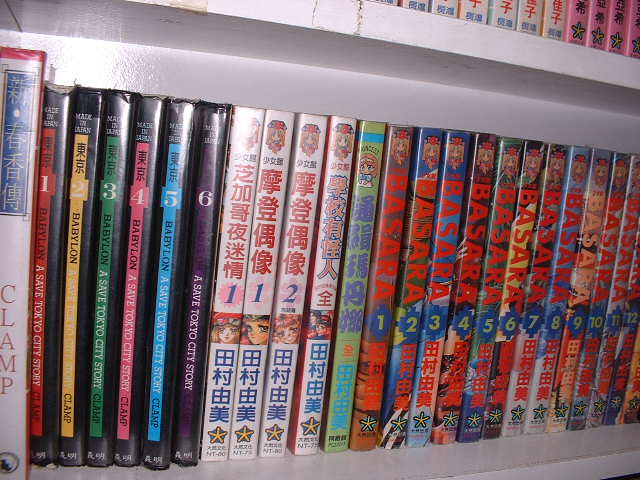The photograph depicts a neatly arranged collection of anime DVDs on a white shelf, with the DVD spines arranged vertically. The visible portion of the shelf showcases a wide array of colorful DVD cases, primarily featuring titles written in Japanese. Prominently, there are volumes 1 through 6 of Clamp Babylon, a series characterized by its black cases. The collection also includes a significant sequence of Basara DVDs, spanning volumes 1 through 12. The Basara series is notable for its vibrant and varied spine designs. Above this shelf, the bottoms of additional DVDs on another shelf are partially visible in the top right corner, hinting at an extensive collection spread across multiple levels. Overall, the image emphasizes a well-organized and visually striking display of anime DVDs labeled with both Japanese and occasional English text.